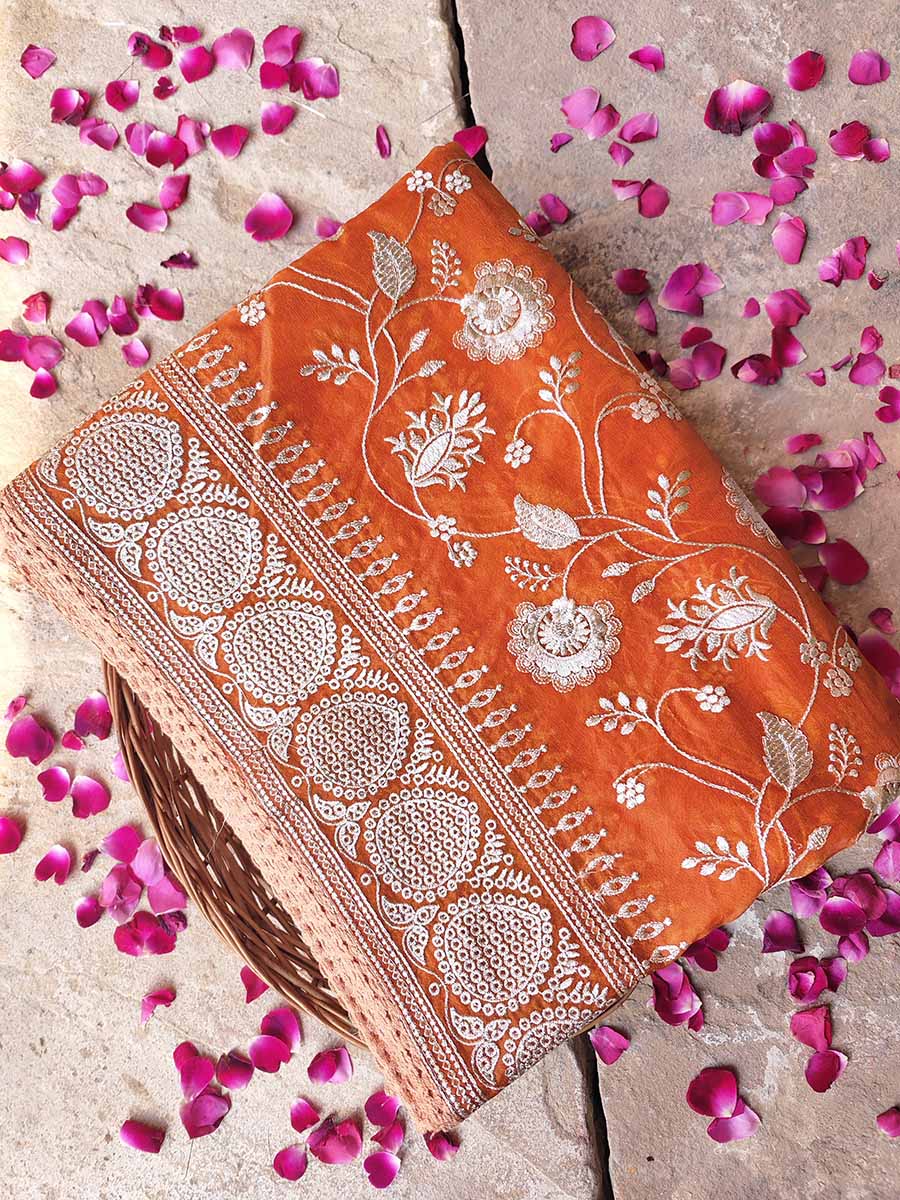The image depicts a vibrant scene where a folded piece of exquisitely bright cloth rests atop a wicker basket. The basket, in turn, is situated on a stone table. The stone table, composed of either a singular slab with a pronounced crease or two adjacent pieces, exhibits a delicate hue of pale grayish-pink. Scattered across the table are loose rose petals in a striking magenta shade, enhancing the visual appeal of the scene.

The cloth, seemingly made of luxurious burnt orange silk, is adorned with intricate white embroidery. The central area showcases an array of different flowers, all interconnected by their stems and leaves, creating a harmonious floral tapestry. Surrounding this central embroidery, the cloth features an elaborate and repeating ornamental border, also rendered in white embroidery, adding to its overall elegance and richness.